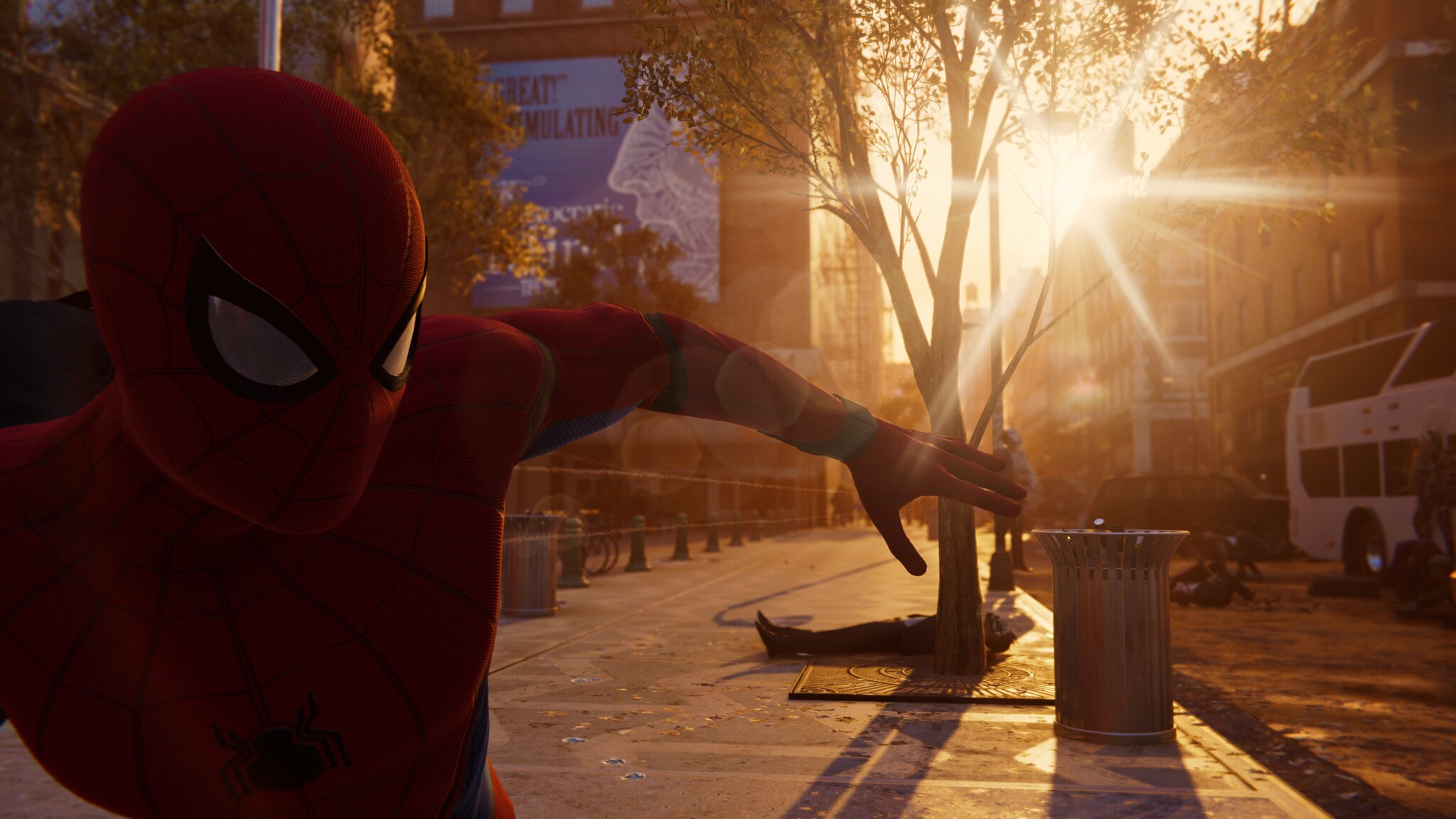The photo features Spider-Man positioned on the far left, set against the backdrop of a bustling city street at sunrise. The early morning light casts a soft glow, making the exact details of the surroundings a bit harder to distinguish. There are trees lined along the sidewalk, just beginning to sprout new leaves, marking the advent of spring. A large bus dominates part of the scene, with someone lying on the ground nearby, creating a sense of recent action or urgency. In the background, buildings rise tall with one displaying a prominent billboard advertisement. Although the scene is somewhat obscured by the glare of the rising sun, the urban environment is palpable, brimming with the energy of a new day. Spider-Man appears as a dark silhouette, blending into the shadows yet unmistakably present, overseeing the city he protects.